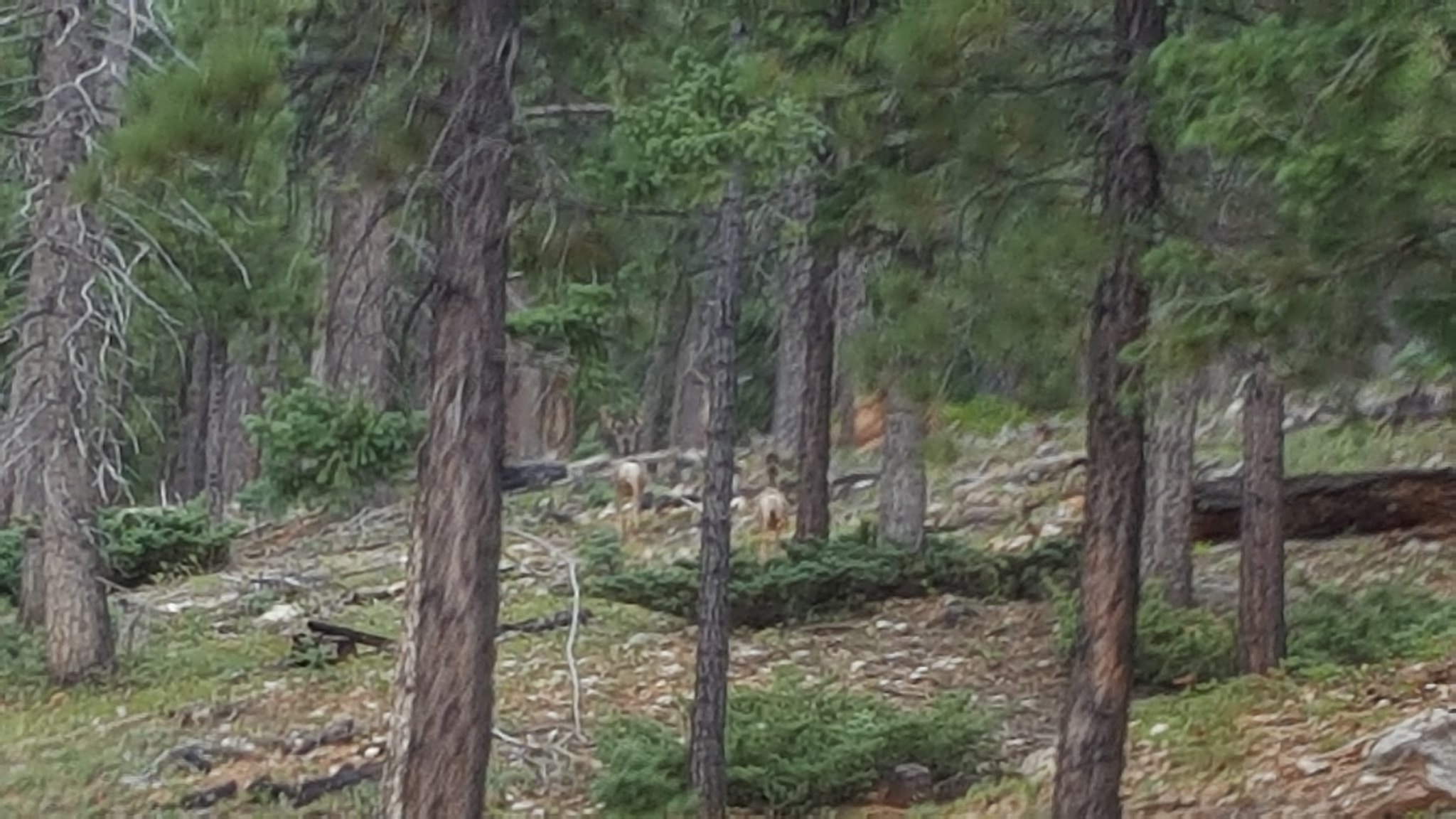The image portrays a dense forest scene with a prominent foreground of tall, slender tree trunks, possibly pine or evergreen trees, many of which have dead lower branches. The trees are closely spaced, extending down a gently sloping, rocky terrain that trends to the left. Scattered across the ground are numerous fallen tree trunks and branches, creating a cluttered forest floor where grasses and low-lying junipers grow. Amidst the tree trunks, two deer are discernible, facing away from the camera, their forms partially obscured and slightly out-of-focus. The background of the image fades into a blur of indistinct foliage, contributing to the overall sense of depth and mystery within this densely packed forest landscape. Additionally, there appears to be an odd, bear-like face near one of the deer, adding an enigmatic element to the scene.